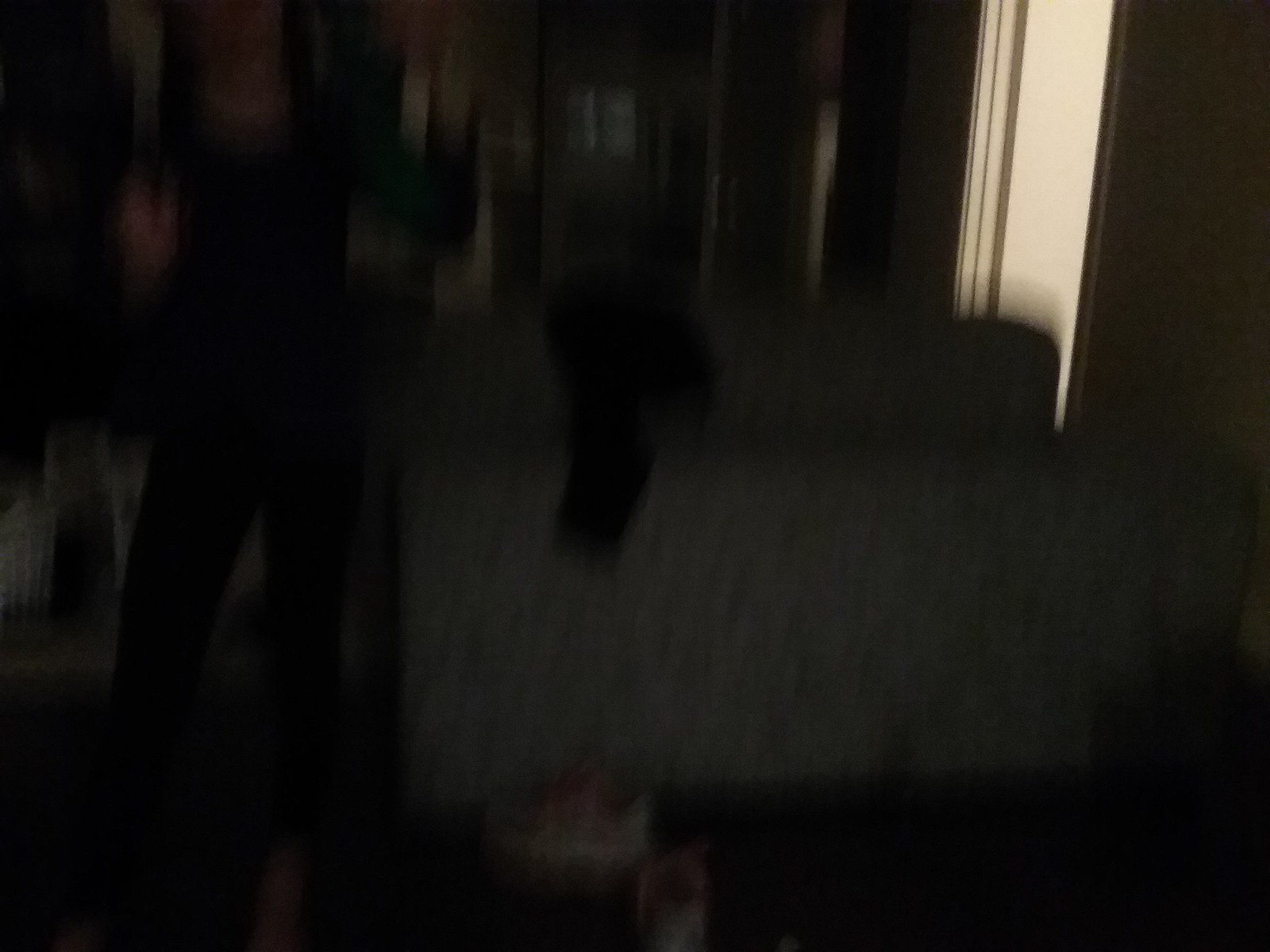A blurry photograph depicts a domestic interior with a focus on a partially imaged person standing towards the left side of the frame. The individual, whose head and feet are cropped out, is attired in a long-sleeved black shirt featuring green splotches near the left arm. Their left hand, fully visible due to a raised and exposed wrist, is lifted to shoulder height, while the right arm is extended sideways just below shoulder level, partially revealing the hand. They are dressed in black long pants and are barefoot. Beside this person on the floor lies a pair of white shoes with pink laces. 

In the background, a blue and blue-green couch faces away from the camera, with a black piece of clothing draped over it. To the further right, a brown cabinet with glass panes, its left door open, is visible. The scene extends to a doorway on the far right, leading into a brightly lit white room, contrasting sharply with the dimly lit foreground. Various items are scattered on a rug positioned on the left side of the image, adding to the lived-in feel of the setting.